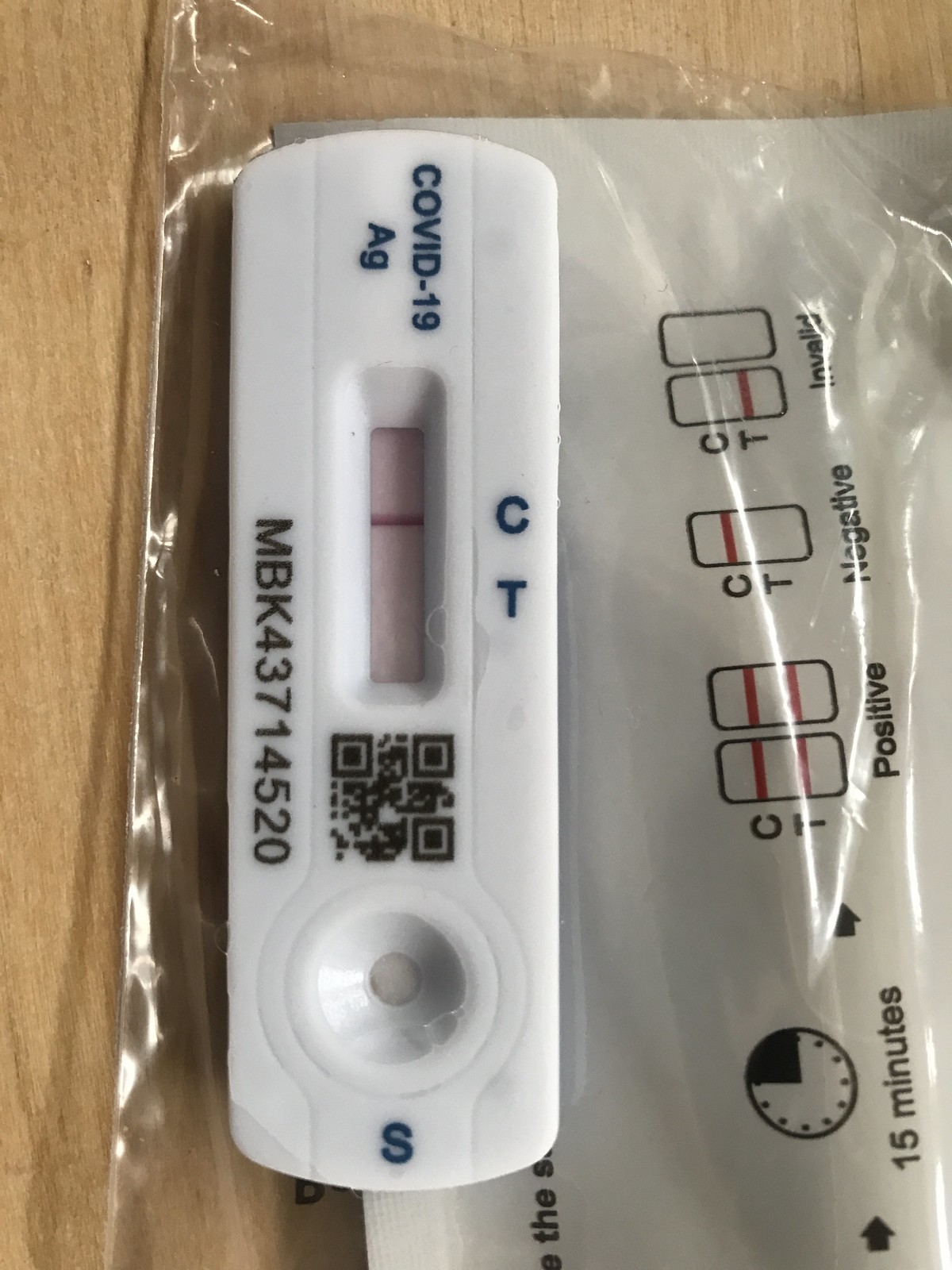The photograph showcases a COVID-19 test kit placed horizontally on a wooden table, viewed from above. The test kit rests atop a transparent plastic bag, which displays printed instructions. The top side of the test faces to the right, while the bottom side faces to the left. The instructions on the bag include a clock icon indicating a 15-minute wait time. It also explains the interpretation of results: two lines below 'C' (Control) and 'T' (Test) indicate a positive result, a single line at 'C' signifies a negative result, and a single line at 'T' denotes an invalid test.

The COVID-19 test itself is a long, white, rectangular device labeled "COVID-19 AG" at the top. Below this label are the letters 'C' and 'T', representing the control and test lines, respectively. The result window currently shows a single line at the 'C' position, indicating a negative test result for COVID-19. Beneath the window, there is a black QR code. At the bottom of the test, there is a letter 'S' adjacent to a circular area with a small hole, which is presumably the sample application spot.